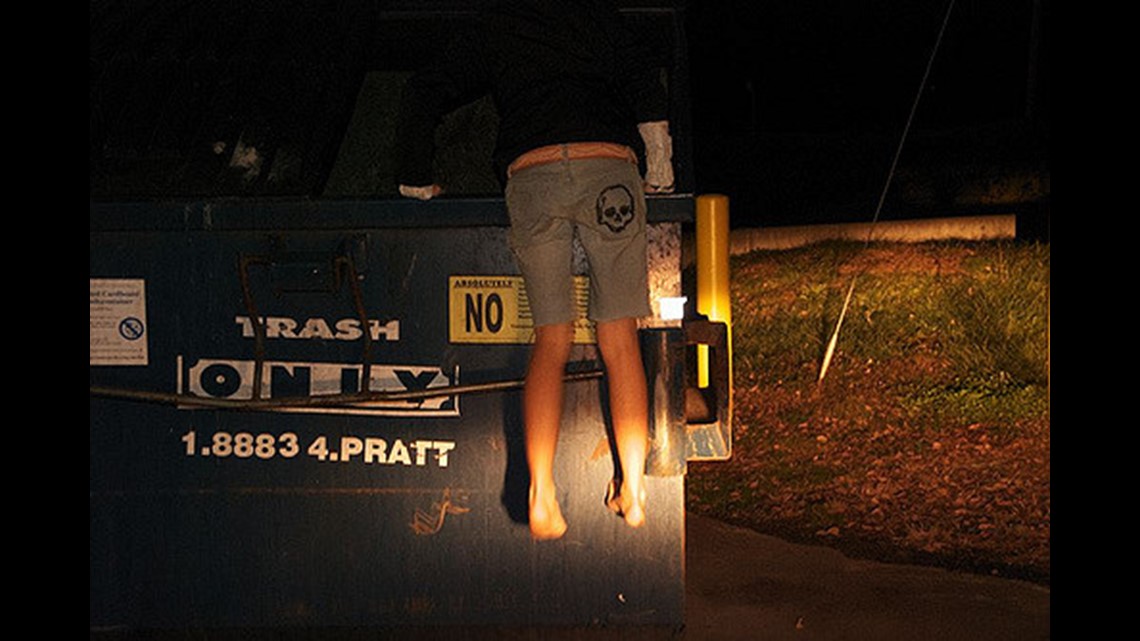In the nighttime image, a man is climbing into a blue dumpster labeled "trash only," with a phone number "1.88834.PRATT" and two additional signs, one white and one yellow with partially visible text. Illuminated by what seems to be car headlights, the scene unfolds outside on a small stretch of pavement bordered by brown dirt and sparse green grass. The man, wearing gray cut-off shorts featuring a skull emblem on the white back pocket and a red belt, is barefoot and has a black shirt layered over a white undershirt with the sleeves visible at the wrists. The upper part of the image is shrouded in darkness, adding to the somber and bleak atmosphere, possibly hinting at the man's desperate circumstances.